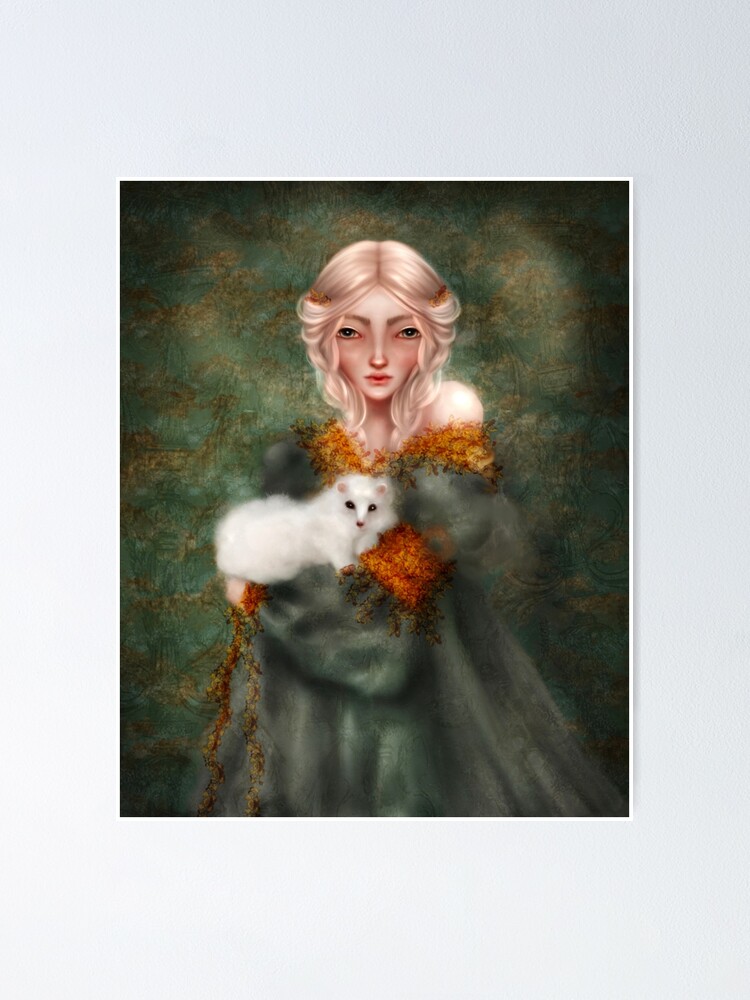The image is a detailed, contemporary surrealistic painting of a woman with a strikingly sad and almost traumatized expression. She has beautiful, short, and pretty blonde hair, reminiscent of Goldilocks, parted in the middle with barrettes on either side that match the orange, red, and yellow fringes of her outfit. Her large eyes are set wide apart on her triangular face. The woman is adorned in a greenish-gray dress, also described as an off-the-shoulders coat or robe, revealing her left shoulder. The dress is embellished with distinctive orange and red fringe around the cuffs and neckline. In her right arm, she cradles an ermine, characterized by its fluffy white body, black eyes, and small pink ears. The background echoes the tones and colors of her attire, blending green, blue, gold, and black in a muted, harmonious pattern that complements the woman's dress and the overall palette of the painting.